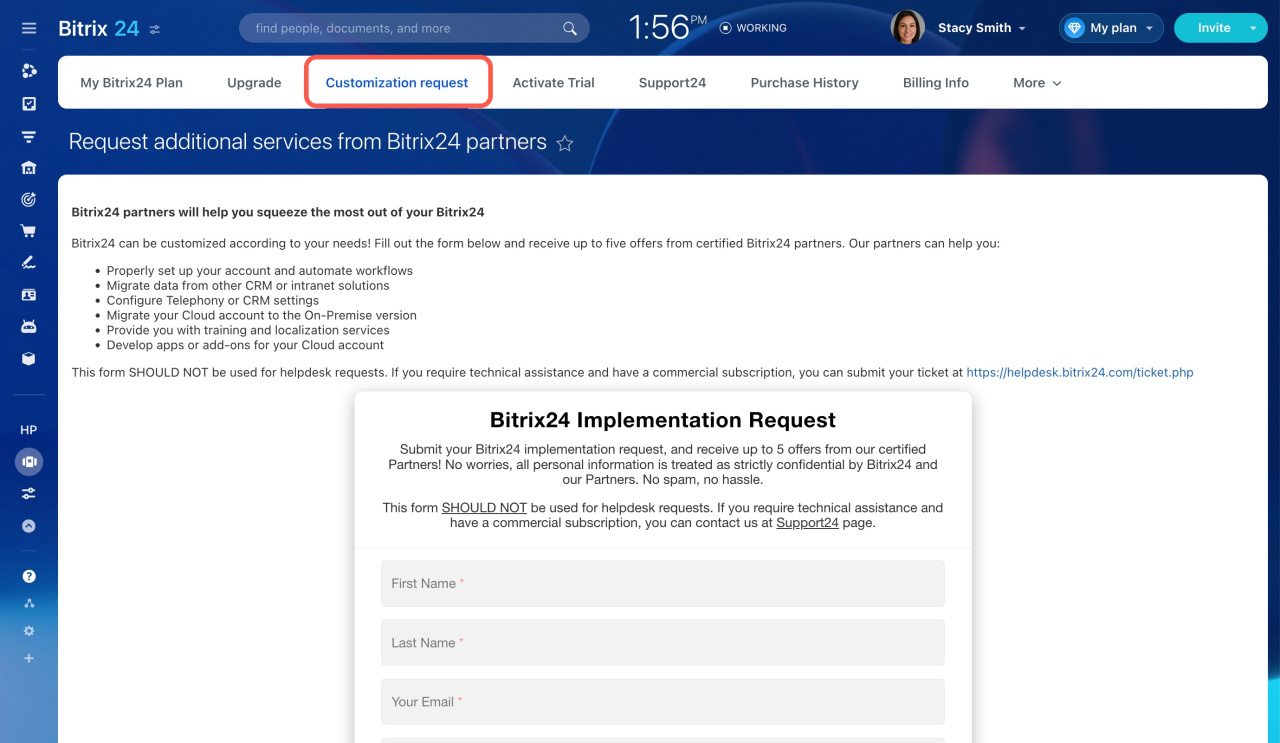The image shows a Bitrix24 web interface primarily dominated by a blue navigation bar at the top. The logo for Bitrix24, spelled "b-i-t-r-i-x" followed by the number "24," is prominently displayed in this blue bar. The bar also contains a search function with suggestions such as "find people, documents, and more." The time displayed is "1:56 p.m."

Beneath the blue bar is a white navigational bar labeled "My Bitrix24 Plan." This bar includes options such as "Upgrade," "Customization Request," "Activate Child Support 24," "Purchase History," and "Billing Info." The "Customization Request" option is highlighted in red.

Below, there is a detailed section headed with "Request Additional Services on Bitrix24 Partners," marked by a star. This section emphasizes how Bitrix24 partners can assist users in customizing their experience. The text states that partners can help with account setup and workflow automation, data migration from other CRM or internet solutions, configuration of telephony or CRM settings, cloud account migration, training, localization services, and developing apps or add-ons for the cloud account.

A note at the end indicates that the form presented should not be used for help desk requests. It advises those with commercial subscriptions requiring technical assistance to submit a ticket through the appropriate website link provided.